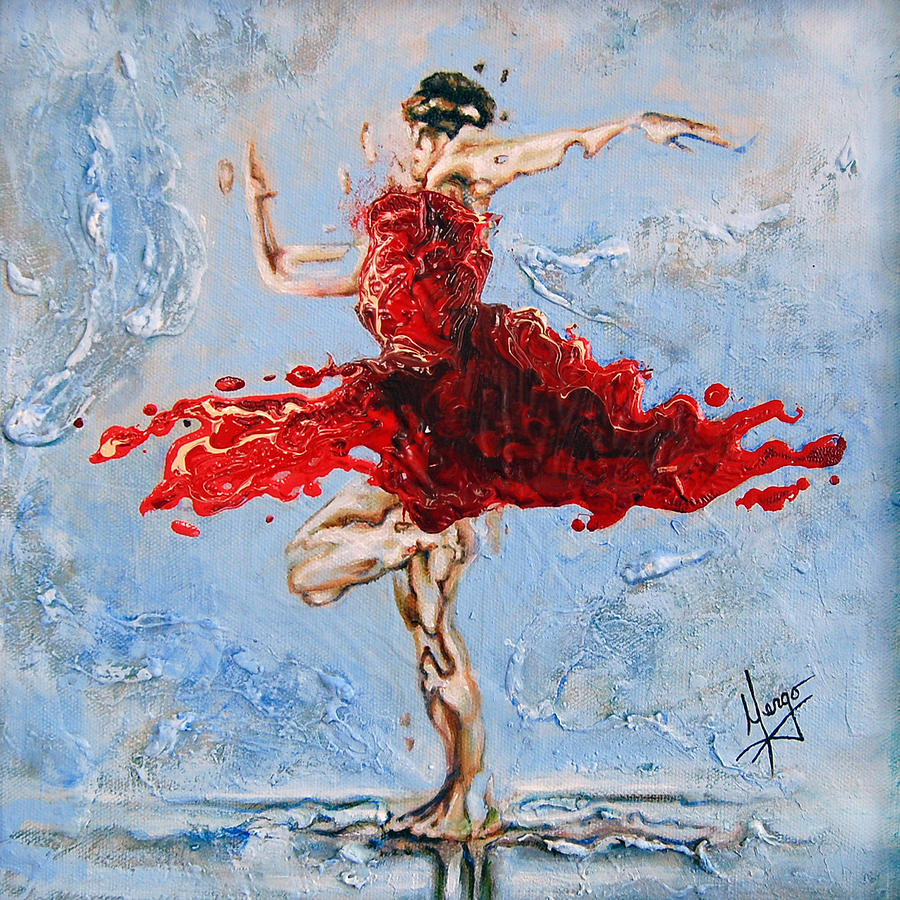This detailed painting captures the dynamic form of a ballerina in mid-motion, adorned in a vivid red dress that appears to flare and swirl around her, giving a strong impression of movement and fluidity. The dancer, with brown hair, executes a graceful pose, standing on one leg with the other leg elegantly raised and bent. Her right arm is lifted at an L-shaped angle while her left arm extends outward, emphasizing the fluidity of her performance. The abstraction of the blue and white background, possibly executed with splashes of watercolor or oil paint, adds an artistic depth to the scene, enhancing the sense of motion and the ethereal quality of the dance. The artist's signature is present but difficult to decipher, potentially reading "Margo" or "Huego." Predominantly, the painting employs colors such as red, light blue, tan, black, and cream, centered attentively on the graceful figure of the ballerina.